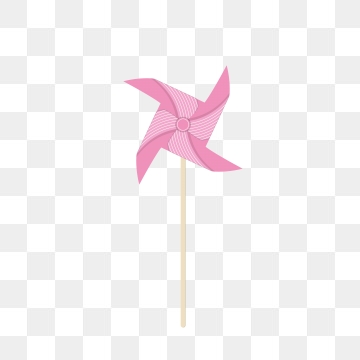The image features a computer-generated gray and white checkerboard background in a perfect 13x13 square grid, indicative of a transparent layer in a PNG file. Dominating the center and occupying about 80% of the image height and a quarter of its width is a stylized, digital pinwheel. The pinwheel has four blades that transition from dark pink to light pink, attached to a beige stick. The overall appearance lacks texture and depth, reinforcing its digital nature. The pinwheel is displayed head-on, centered against the static checkerboard background, clearly emphasizing the product in isolation.